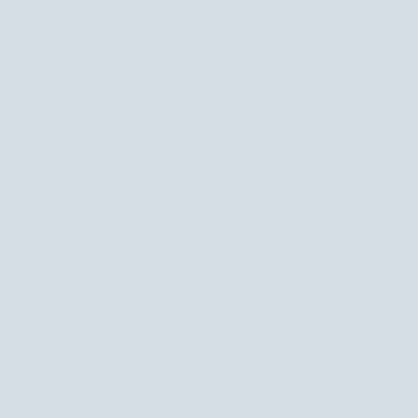The image features a light gray background that distinctly stands out from plain white, indicating a deliberate choice to maintain a neutral, yet subtly contrasting shade. There are no additional elements or text overlaying the gray backdrop—no website banners, no application icons, no time stamps in the corners, nor any login or enter buttons that might typically be seen in such contexts. It is a clean, uninterrupted field of light gray, devoid of any distinguishing marks or focal points, presenting a minimalistic and uncluttered visual frame.